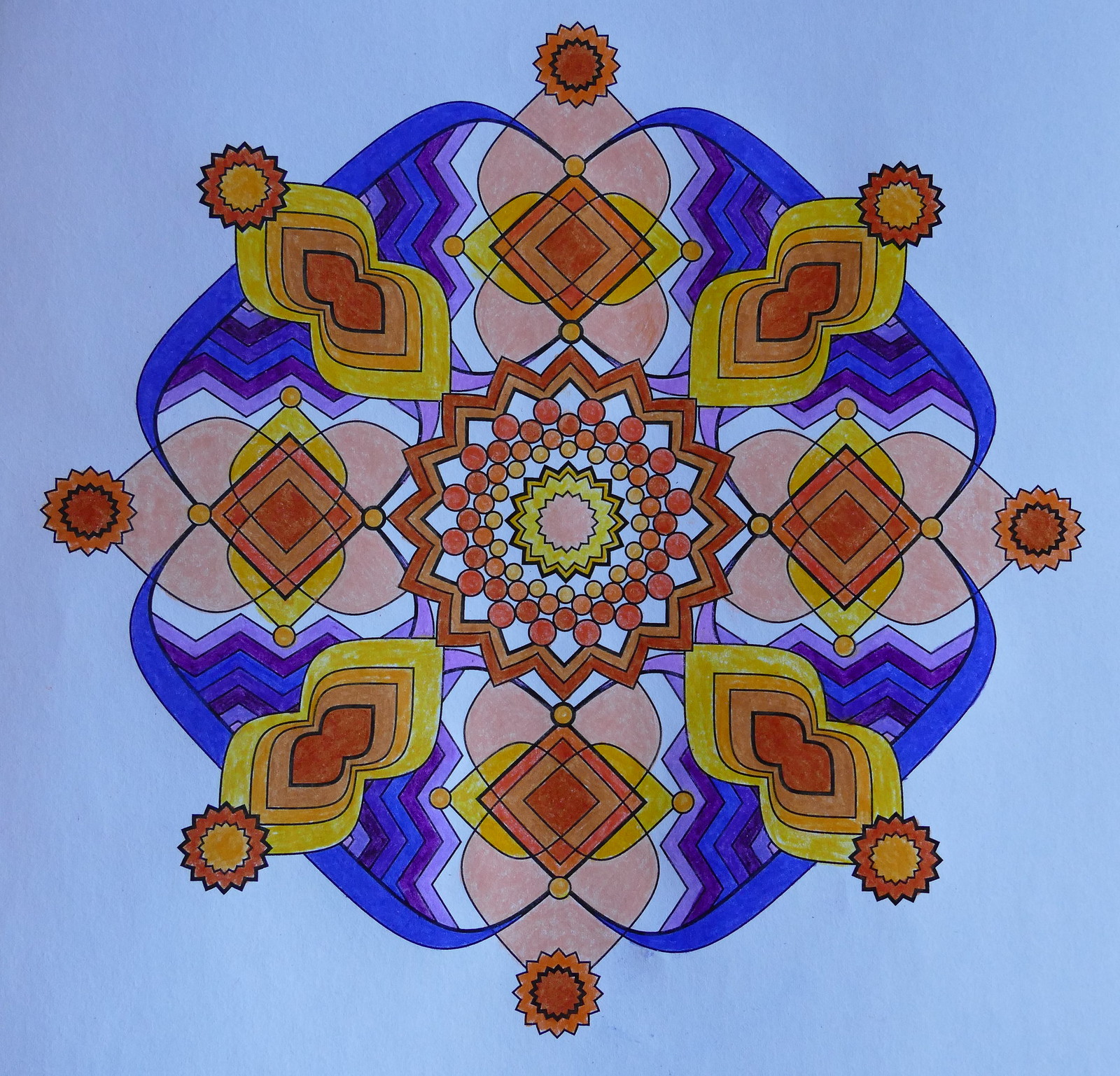The image features a highly zoomed-in view of a hand-drawn artwork on an indeterminate white surface. Positioned centrally in the frame are intricate geometric patterns consisting of various shapes and colors. Among these patterns are circles resembling mini suns, characterized by intricate zigzag lines radiating outward. Some suns have an orange core encircled by black outlines and orange zigzag rays, while others showcase a yellow core with orange zigzags. The artwork further features an array of shapes, including orange-colored circles and both yellow and orange diamonds. Additionally, zigzag lines in a spectrum of colors—purple, blue, and white—are interspersed throughout the design, adding to its complexity and dynamism. The lack of visible edges or contextual surroundings focuses attention solely on the vibrant and elaborate patterns within the drawing.